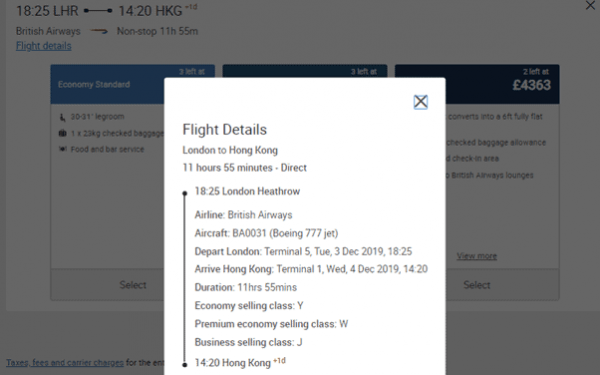This image is a screenshot of a website page featuring a detailed pop-up card. The pop-up card appears in the upper right-hand corner and includes an "X" button to close it. 

On the left side of the card, it lists the following flight details:

- **Flight Route**: London (LHR) to Hong Kong (HKG)
- **Duration**: 11 hours and 55 minutes, direct 
- **Departure Time**: 18:25 from London Heathrow on Tuesday, December 3rd, 2019
- **Arrival Time**: 14:20 at Hong Kong Terminal 1 on Wednesday, December 4th, 2019
- **Airline**: British Airways
- **Aircraft**: Boeing 777
- **Terminal (London Departure)**: Terminal 5
- **Travel Classes**:
  - Economy (Selling Class Y)
  - Premium Economy (Selling Class W)
  - Business (Selling Class J)

In the original screen's upper left-hand corner, the flight details are summarized: "18:25 LHR – 14:20 HKG, British Airways, non-stop, 11:55." Below this summary, there is a clickable link labeled "Flight Details," which, when clicked, brings up the detailed white pop-up card.

This detailed caption provides a thorough description of the content and layout of the website page and its pop-up card.